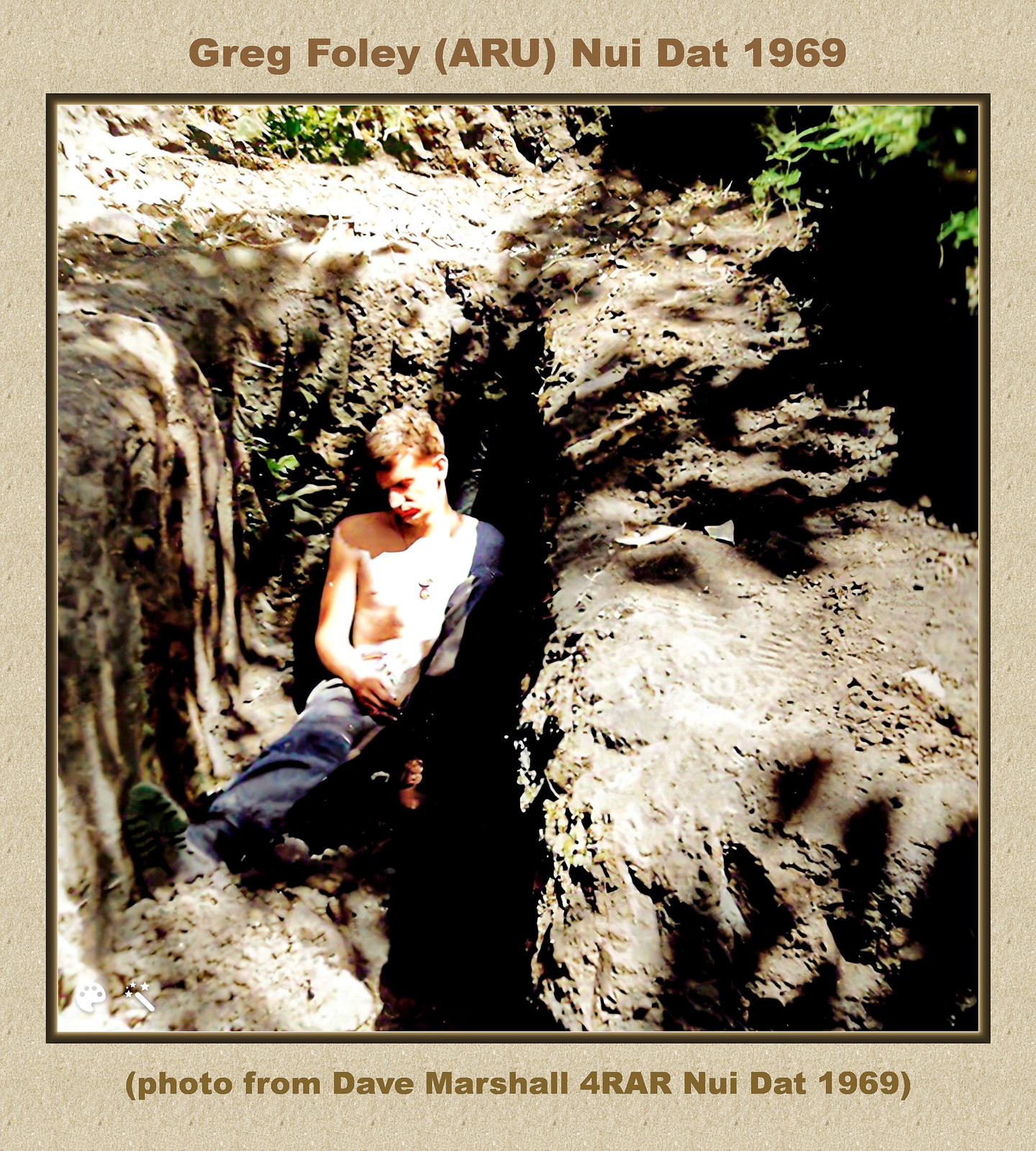The photograph, slightly taller than it is wide and printed on pebbly light gray cardstock, captures an intense moment during the Vietnam War. At the top of the image, text reads "Greg Foley, ARU, Nui Dut, 1969," and the bottom notes, "photo from Dave Marshall, 4RAR, Nui Dut, 1969." The central image, surrounded by a black border, reveals a young, shirtless Caucasian male with short reddish hair, wearing jeans and a necklace, sitting in a narrow, grave-shaped dugout approximately four to five feet deep. The gray earth walls of the hole blend with the pebbly background, while sparse green vegetation peeks from the edges, suggesting a swampy terrain. The man's head is angled downward, perhaps indicative of sleep or exhaustion amidst a tense environment. Above him, a tangle of trees, grass, and bush contrasts with the stark grayness of the earthen dugout, hinting at both cover and confinement. The image poignantly depicts a soldier's moment of reprieve or vulnerability during a turbulent time.